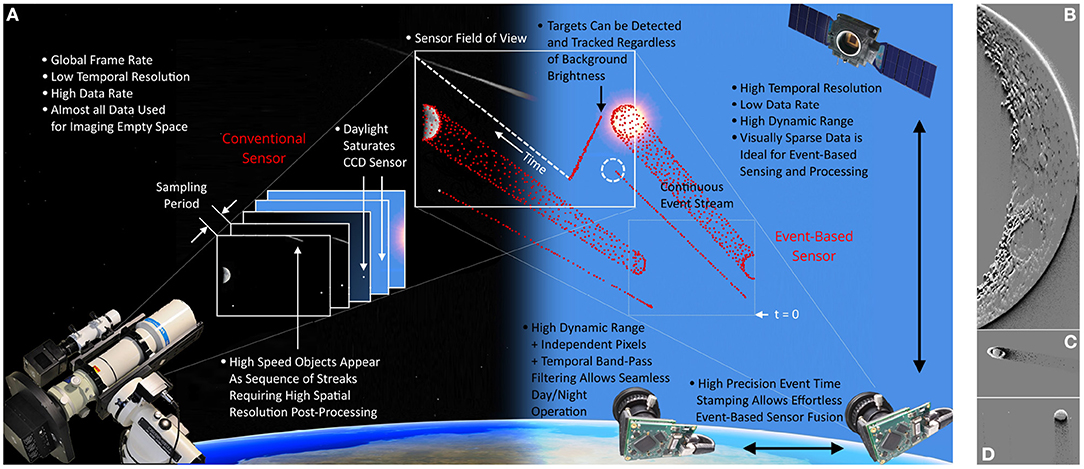The image is an intricate, horizontally oriented illustration, resembling a page from a scientific textbook. The illustration is slightly blurry, making some of the text difficult to read. On the left side, the main section labeled with a capital "A" encompasses the majority of the space and contains multiple schematics. This section features a high-powered professional telescope, pointing upward to the right, with its various parts labeled in a combination of white, black, and red text. Superimposed on this illustration is a real photograph of the telescope, highlighting its significant role in capturing high-resolution images. 

On the right side, separated from the main image by a vertical white strip, are three black and white images, labeled "B," "C," and "D." Image B is the largest, with C and D being of equal size. These smaller images, possibly negative or texture maps, demonstrate the high spatial resolution post-processing capabilities of the system.

The bottom left of the image shows the curvature of Earth, with sections depicting land and water. High dynamic range and temporal bandpass filtering are noted features, enabling seamless day-night operation and target detection regardless of background brightness. The top right corner of the image contains a depiction of a satellite, indicating the principles of the sensor's field of view and the mechanisms of the telescope and the CCD sensor.

Overall, the image is a comprehensive diagram detailing the use of telescopes and satellites in capturing and processing high-resolution photos from space, illustrating the interconnectedness of various scientific principles and photographic technologies.